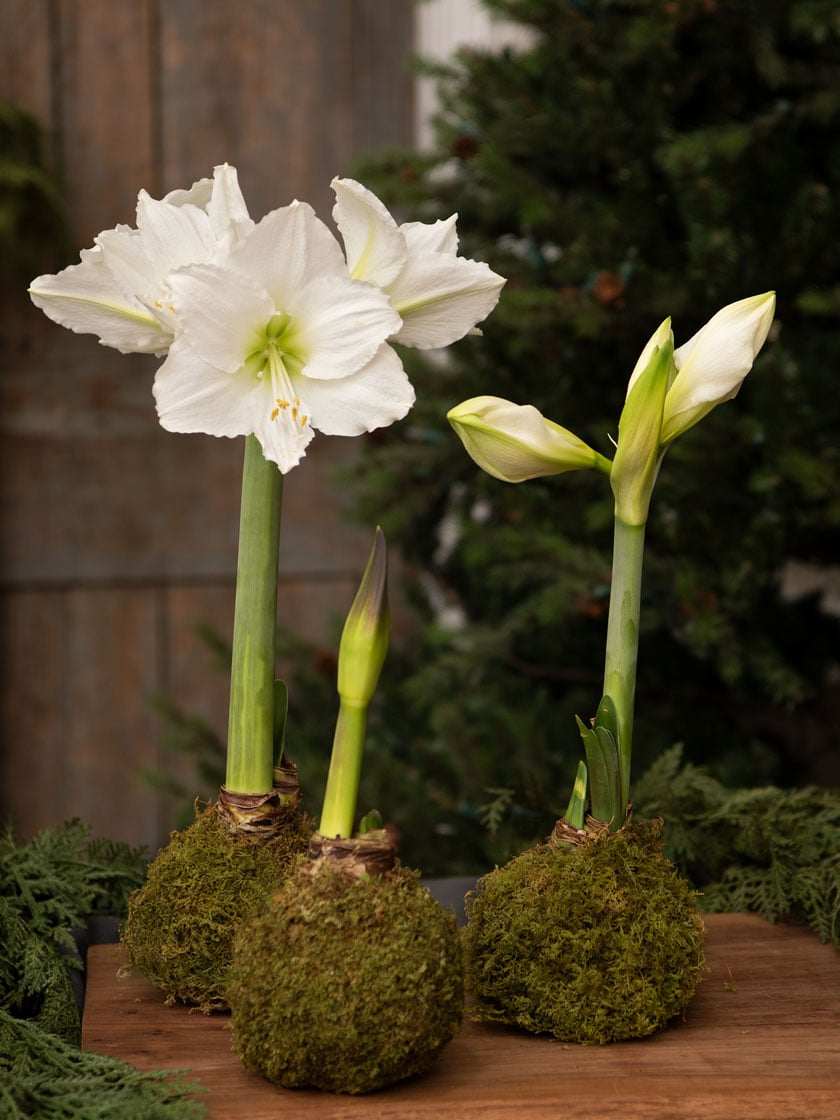The image depicts a trio of flowers situated on an unpolished wooden table outdoors. Behind this rustic arrangement, there's a wooden wall with out-of-focus trees and lush vegetation providing a natural backdrop. Each flower is embedded in a moss-covered, baseball-sized bulb resting on the table, displaying various stages of blooming. 

Starting from the left, the first flower has fully bloomed, showcasing large, oval, flat white petals arranged in a triangular pattern with smaller inner petals and visible interior parts. The central flower sports a tall green stalk tapering to a dark gray point at the top, where it is just beginning to develop a flower. The bloom remains closed and green, hinting at its imminent opening. Finally, the flower on the right shows three buds at the top of its stalk, with two of them transitioning from green to white and appearing close to blooming, while one remains tightly closed. The earthy moss and soil base of each plant further accentuate the natural, unrefined aesthetic of the scene, making the flowers the focal point of this serene outdoor setting.